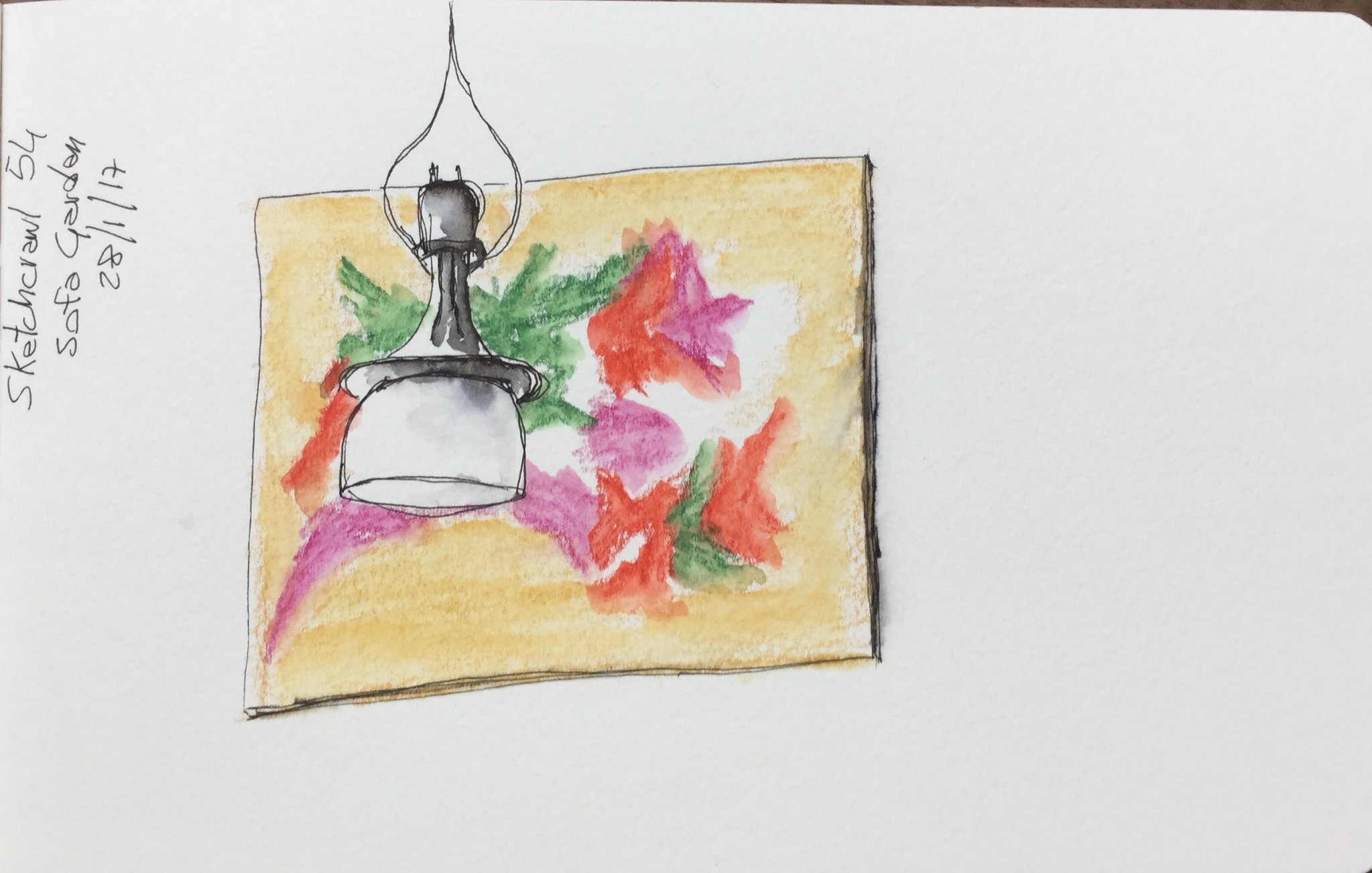The artwork is a detailed illustration on white paper or cardstock with a focus on a central, slightly three-dimensional yellowish-tan rectangle, adorned with somewhat abstract floral designs featuring red, pink, and green elements that appear blurry or stylized. In front of this rectangle, there's a hand-drawn light fixture in black, gray, and white tones, resembling a ceiling-hung lantern with a chain or wire connecting it to the unseen ceiling. The light fixture includes an opaque glass shield, obscuring any depiction of a lightbulb. To the left of these central elements, the handwritten text reads, "Sketch Crawl 54 Sofa Garden," alongside a date written in European format, "28-1-17," suggesting a significant event or session related to this artwork. The background remains predominantly white, providing a stark contrast and focus on the artistic elements depicted.